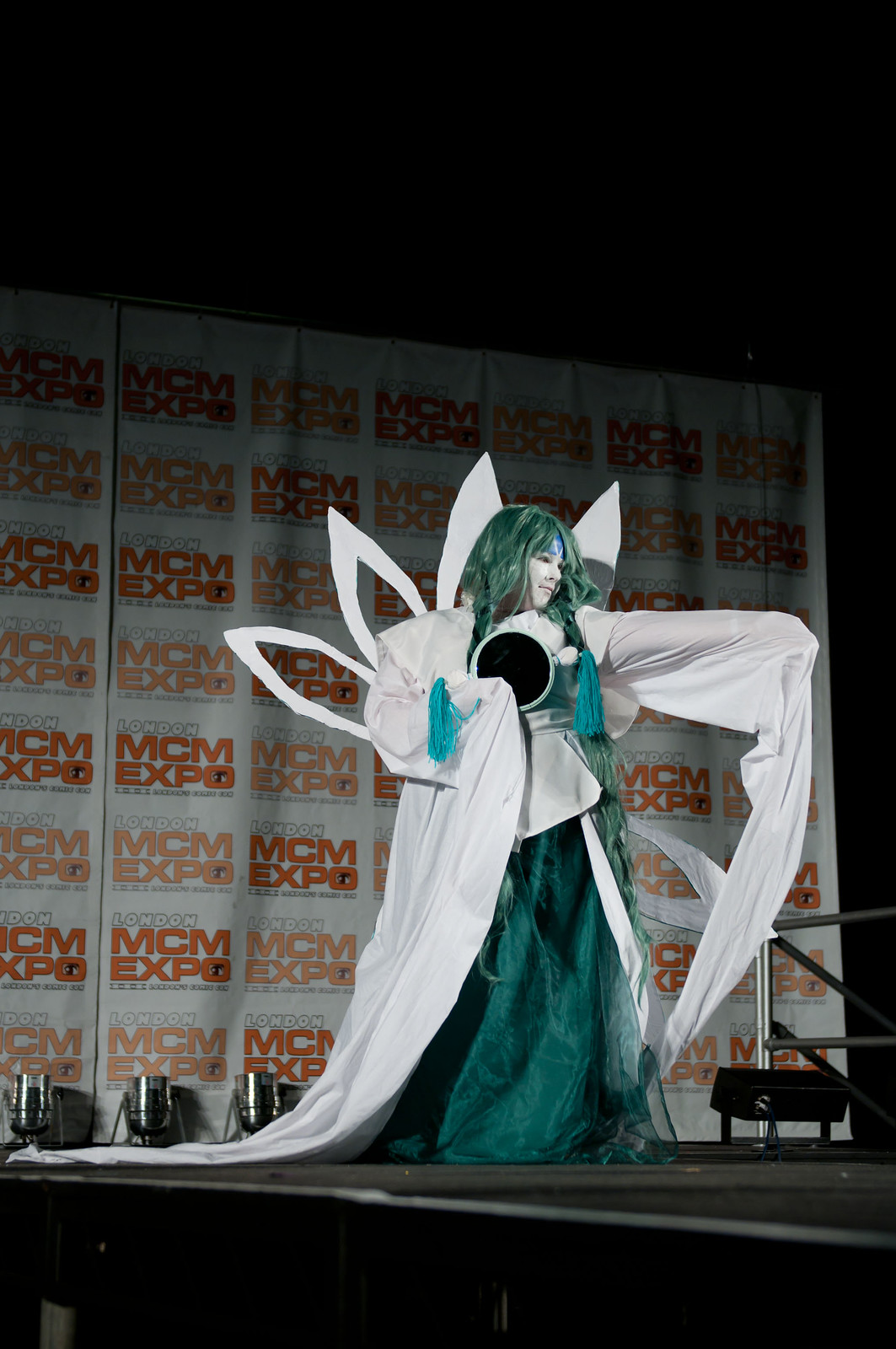In this captivating image, we see a cosplayer immersed in character, standing confidently on a dark stage at the London MCM Expo. She is adorned in an elaborate costume featuring a floor-length, emerald green dress coupled with a flowing white robe. This robe cascades into long, ghost-like sleeves that gracefully trail to the floor, adding an ethereal quality to her appearance. Enhancing the ensemble, greenish-blue tassels dangle near her wrists. Her striking green hair and face painted white further enhance her transformation, while petal-like spikes or wings extend from her back, contributing to the fantasy element of her costume. She stands with her left arm raised, pointing outward, and holds a round object in her hand. Behind her, a substantial advertisement wall prominently displays the 'MCM Expo' logo repeatedly in various shades of orange, cementing the setting as an energetic expo environment.